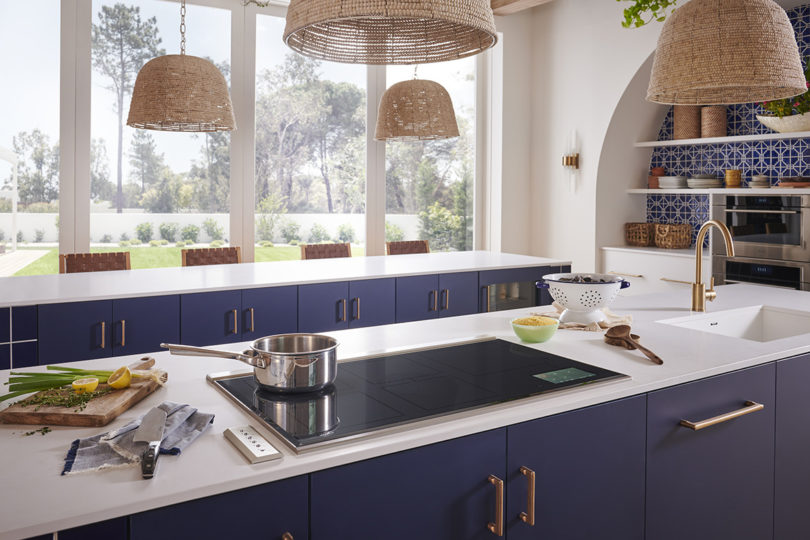This vibrant and detailed kitchen photo captures an inviting space bathed in daylight. The kitchen boasts four expansive, clear windows that offer a picturesque view of green grass and several distant trees, illuminating the room with natural light. The countertops are white with blue cabinets below, adding a fresh and clean aesthetic.

On the left side of the kitchen, there's a wooden chopping block featuring halved lemons, celery, leeks, and green onions, with a knife set on a towel beside it. Central to the layout is a black electric stovetop, adorned with a steel pot. To the right of the stovetop, the countertop extends, hosting bowls and spoons, transitioning neatly into a brass sink at the far end.

The kitchen design includes two functional islands—one dedicated to food prep and the other designed for casual dining, accompanied by four seats partially visible above the counter. The space is elegantly lit by brown stick lamps suspended from the ceiling. Additionally, the kitchen features a beverage refrigerator and integrated ovens, enhancing its modern appeal. Overall, this spacious and well-appointed kitchen evokes a sense of contemporary, functional charm.